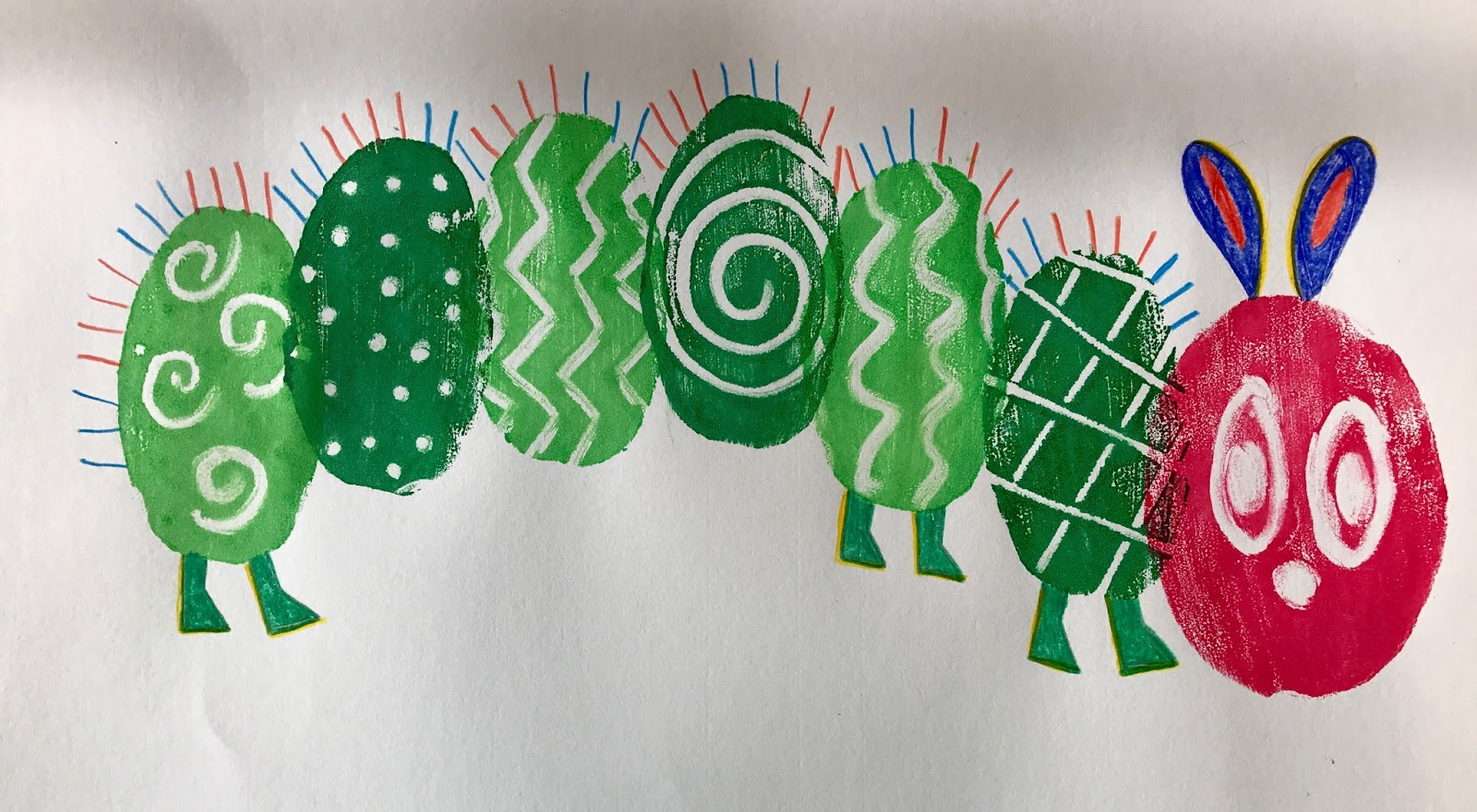This image showcases a colorful caterpillar likely drawn or crafted by children, possibly as part of an elementary school project or the cover of a children’s book. The backdrop is a light white with gray shadows, giving a clean canvas for the vivid creation. The caterpillar itself features a vibrant red head adorned with expressive white eyes and prominent blue ears outlined in yellow with red centers. Its body is composed of six oval-shaped green segments, varying between light and dark green, each embellished with unique white patterns, such as curly lines, dots, squiggles, concentric circles, and crosshatches. Each segment has tiny red and blue spikes protruding from short indents along the top. Notably, the caterpillar has three pairs of green feet—two pairs on the first body segments and one pair on the last, though real caterpillars typically have more legs. This delightful and colorful artwork stands out against its simple background, showcasing the creative imagination of its young artists.